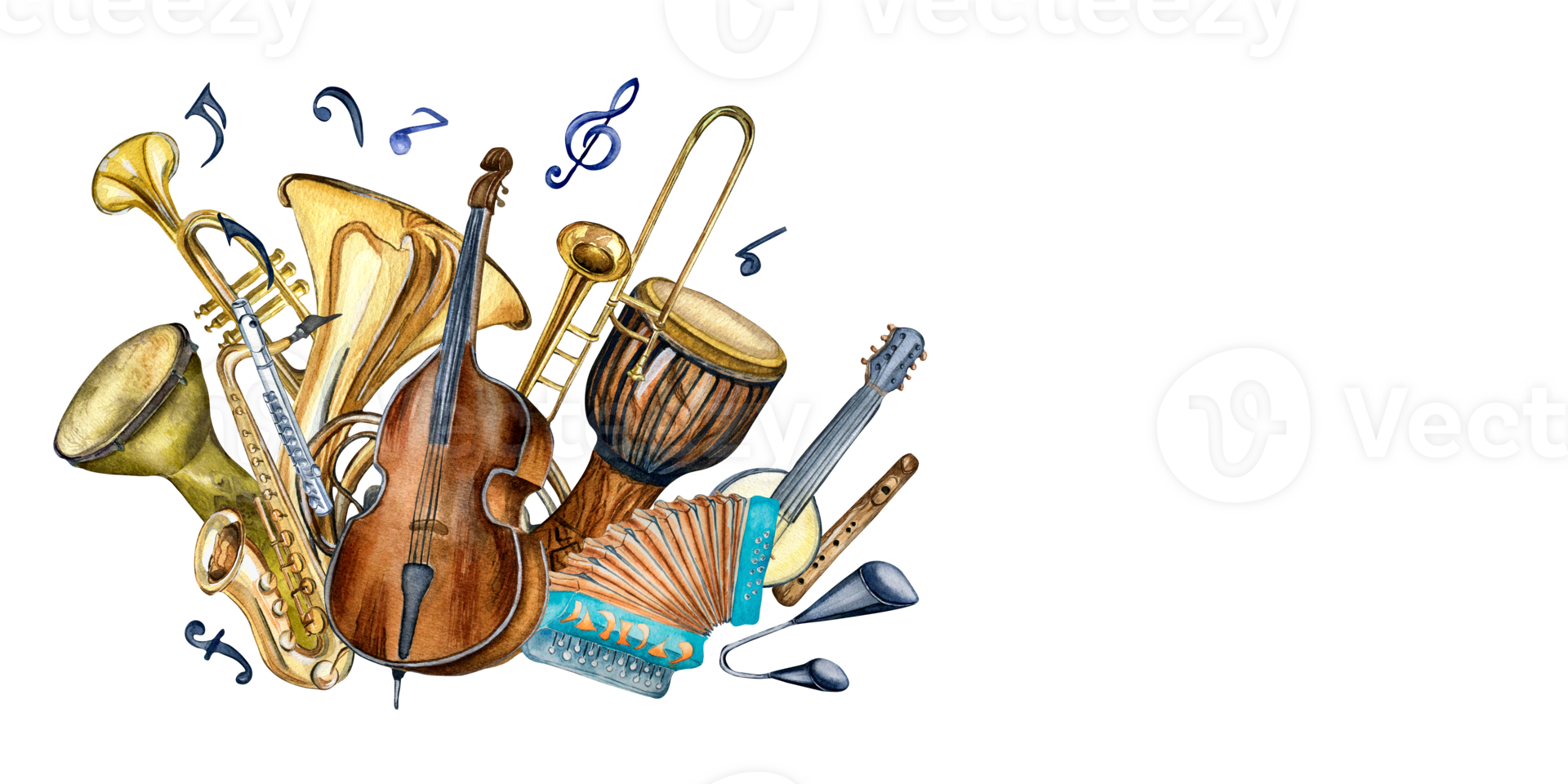This vibrant drawing features a diverse collection of musical instruments, artfully arranged and colorfully depicted. On the left side, there are several wind instruments including a gold-colored saxophone, a trumpet, and a trombone, alongside a large C-shaped tuba. Toward the center of the image, a dark brown cello or violin stands prominent, partially overlaying a drum with a light tan top and a shiny dark wood base accented with black lines. An accordion and a banjo, adorned in varied hues, appear nearby.

To the right, among the more conspicuous items, are another trumpet, a drum, a ukulele, and a mysterious instrument resembling two cups connected by a cord. A flute or recorder lies nearby, contributing to the rich assortment. Scattered across the scene are numerous musical notes and symbols, primarily in shades of blue, with one symbol near the saxophone resembling an F.

The instruments boast a palette of golds, browns, blues, pinks, and yellows, creating a lively and engaging composition. The artistic medium appears to be drawn or painted rather than photographed, with no people or text present, highlighting the instruments and musical symbols as the sole focus.